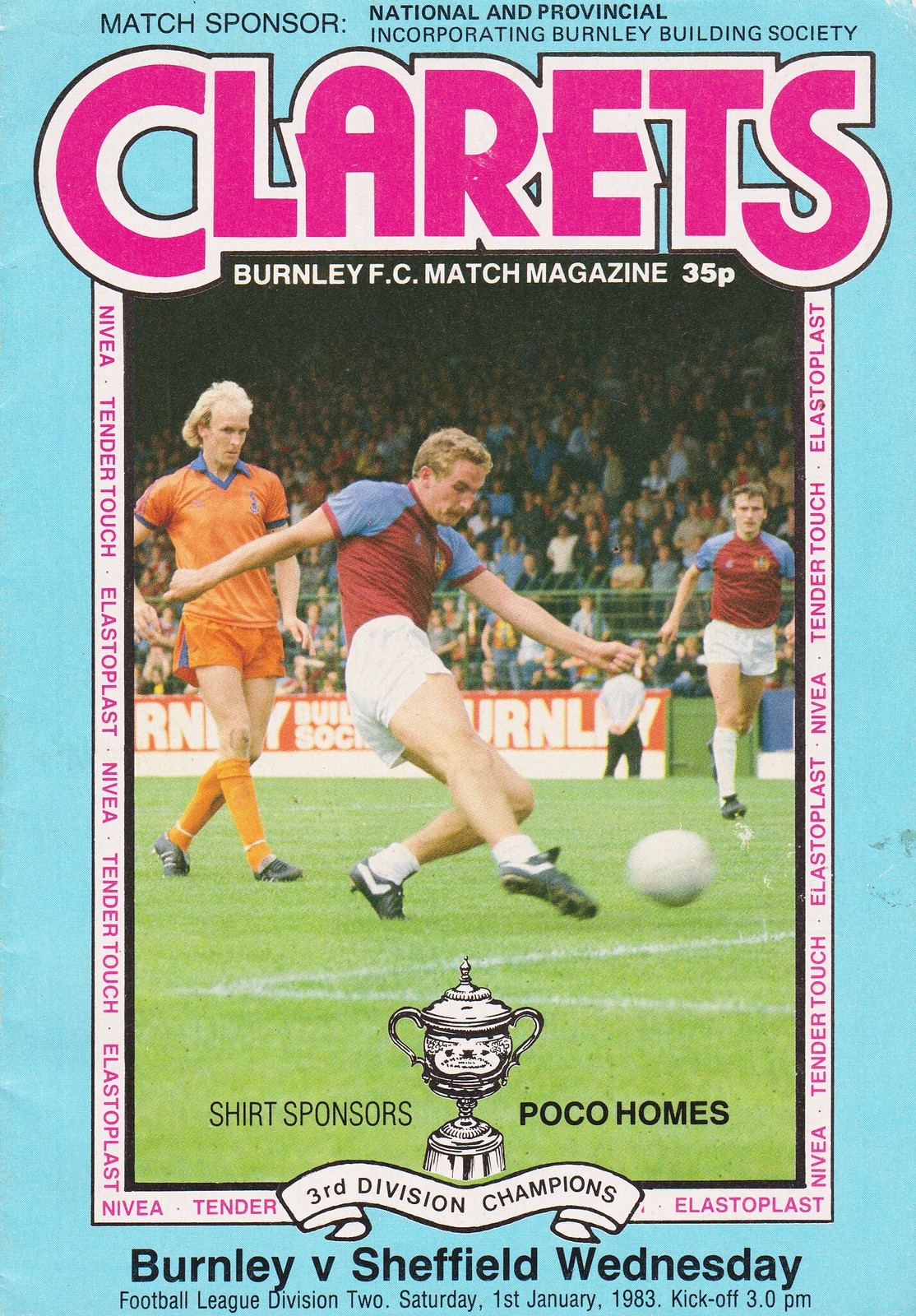This image is a tall, rectangular poster with a bright blue background. At the top, it prominently features the word "CLARETS" in large, bright pink capital letters, outlined first in white and then in black. Below this title, there is a vertical rectangular photograph capturing a dynamic soccer scene. In this photograph, players are in the midst of a match: two athletes are clad in red and blue uniforms while another on the left sports an orange and blue kit, all situated on a lush green field with an audience in the background. The action shot is framed by a white border adorned with capitalized pink text. At the bottom of the poster, a white ribbon bears the inscription "Third Division Champions." Further below, in bold black lettering, the match details "Burnley v. Sheffield Wednesday" are displayed. Additional information notes that this is a program for a soccer game, specifying the event as the Football League Division II match on Saturday, 1st January 1983, with a kickoff at 3 p.m., sponsored by the National and Provincial Incorporated Burnley Building Society.